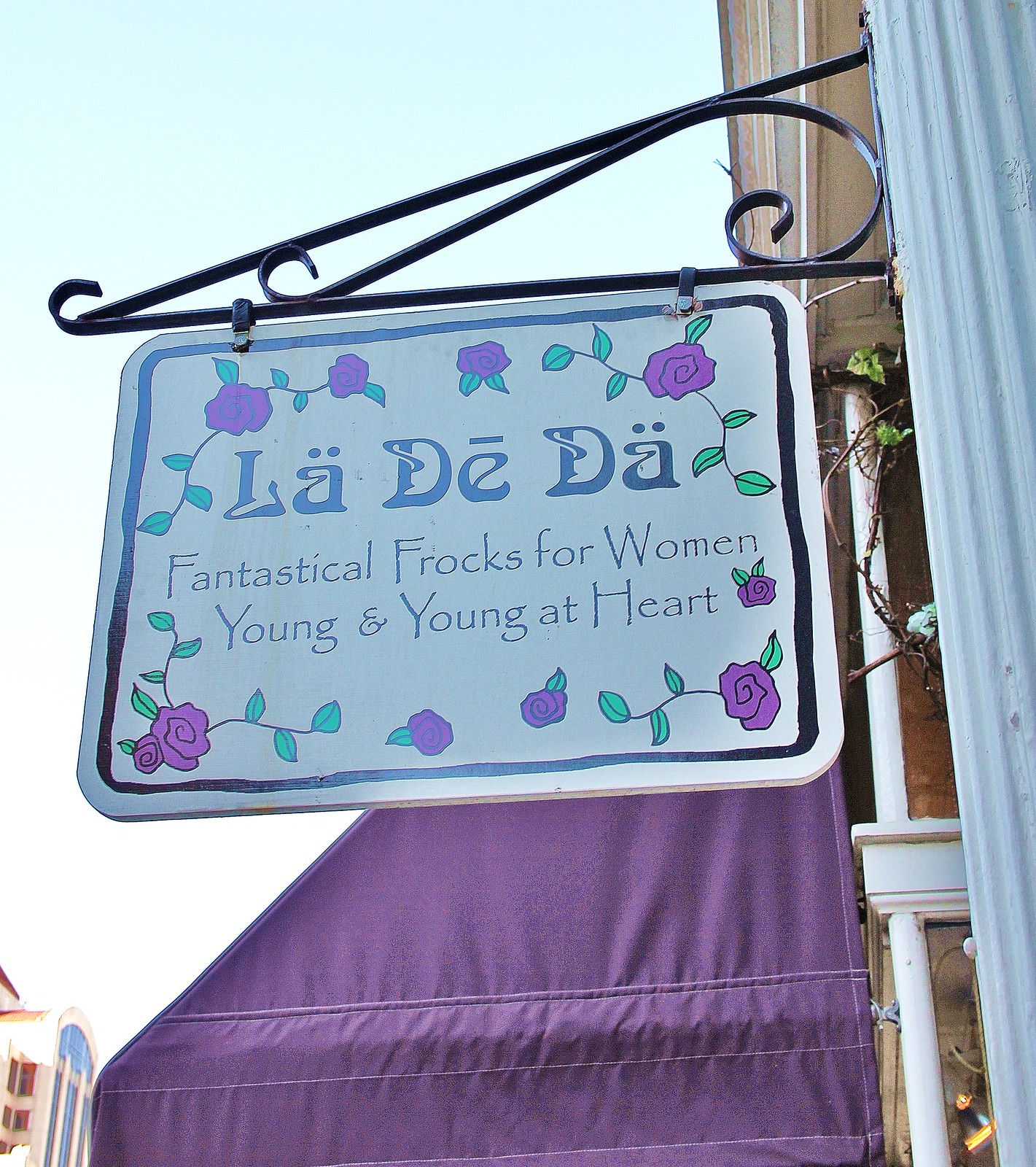This image, taken outdoors during daytime, captures a detailed side view of a charming building. Dominating the scene is a white sign with a black rectangular border, hanging from a black metal arm extending at a 90-degree angle from a white column. The sign, embellished with bevelled edges and delicate purple flowers intertwined with green vine-like leaves, reads, "La-De-Da, fantastical frocks for women, young and young at heart." Below the sign, a purple awning seamlessly matches the hue of the flowers. The awning, viewed from the side, highlights the sunlight illuminating the scene without showing the sun. The right edge of the image features a white beam and column, with tree branches and green leaves visible in the background, alongside a glimpse of a building across the street characterized by red flags, blue windows, and red shutters.